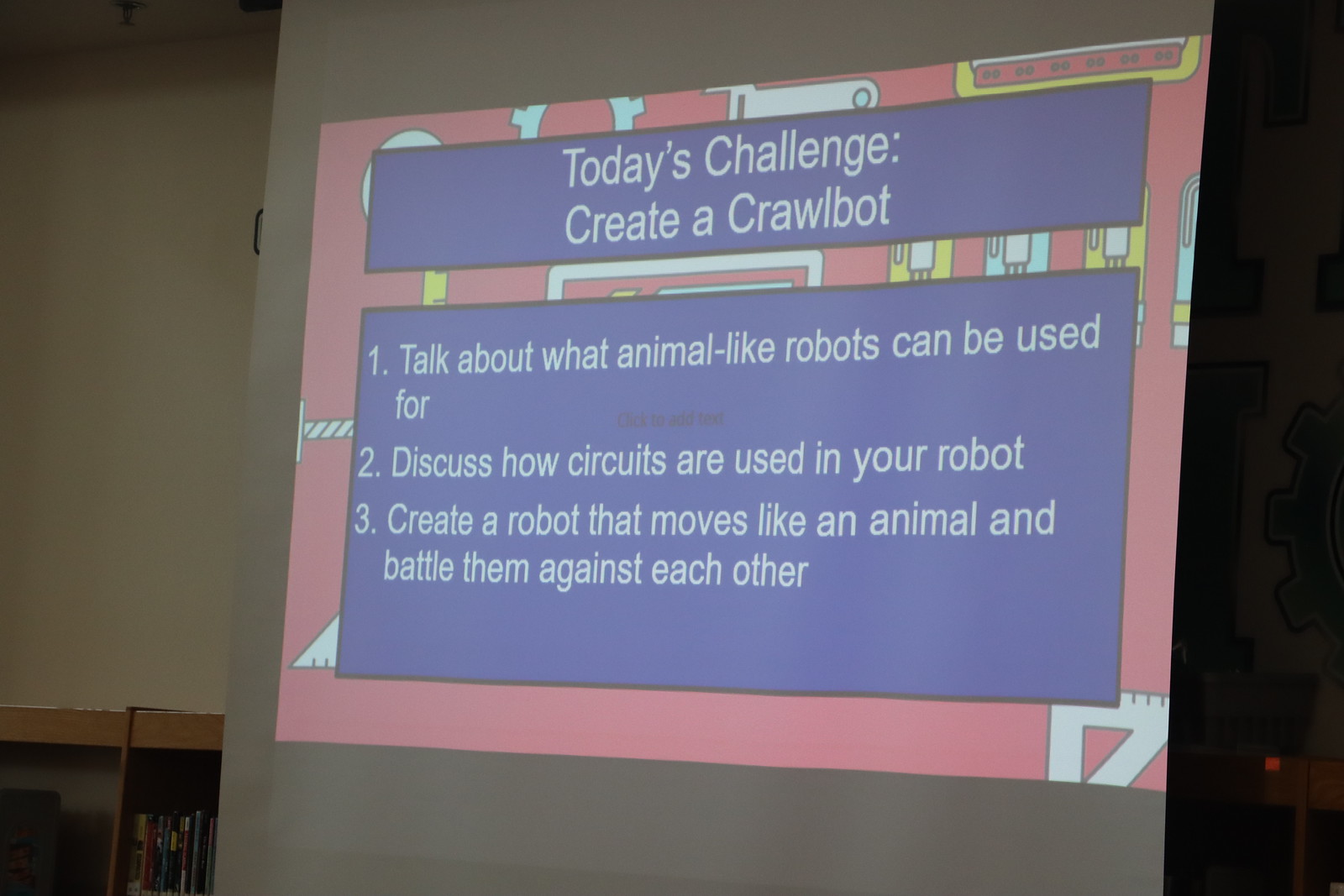The photograph captures a presentation slide projected onto a white screen. The slide features a prominent red background with a digital pattern in white, resembling a circuit board. Central to the slide are two blue rectangles. The top rectangle, inscribed with white text, reads "Today's Challenge." The bottom rectangle outlines a three-part task as follows: 

1. Talk about what animal-like robots can be used for.
2. Discuss how circuits are used in your robot.
3. Create a robot that moves like an animal and battle them against each other.

Notably, the image contains no people or additional items, solely focusing on the detailed and colorful slide content.